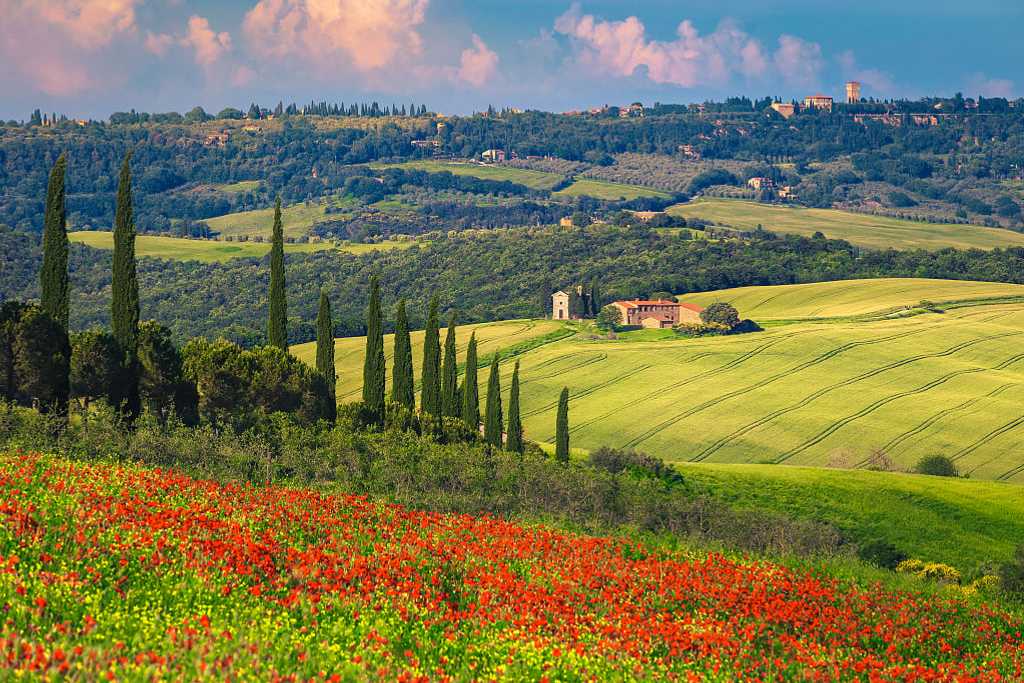The photo captures an expansive, picturesque outdoor scenery. In the foreground, a vibrant field of red blooming flowers with lush green stems stands out prominently. As the eye moves further, it transitions into green grass, dense bushes, and tall, slim arborvitae trees forming a natural wall. Beyond this, manicured fields and a well-maintained landscape reveal themselves, highlighting a large, brown house with a red roof and a tall, smaller building beside it in the distance. To the right, additional buildings peek out. The backdrop features more clear fields, interspersed with woods and trees, and extending to the horizon where more structures are faintly visible amidst the greenery. The sky above is a serene blue, adorned with pink clouds, adding a touch of magic to the idyllic scene.